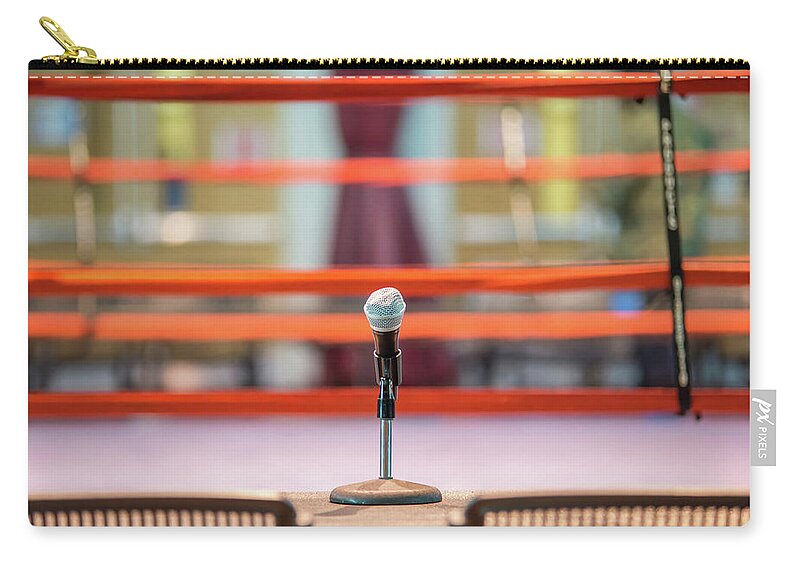The image depicts a computer-generated photograph printed on a small personal wallet or coin purse, characterized by a distinct golden zipper situated at the upper left. The central feature of the photograph is a short black microphone with a silvery head, mounted on a circular, flat gray base. The microphone appears to be the focal point of the image. Surrounding the microphone, the background is notably blurry and includes several horizontal red lines, reminiscent of ropes from a boxing ring, with blurred colors of purple, white, and gold interspersed. Additional details in the image include the partial, blurred views of two wooden chair tops positioned at the bottom left and right corners. On the right side of the wallet, a gray and white tag with the text "PX Pixels" is visible.